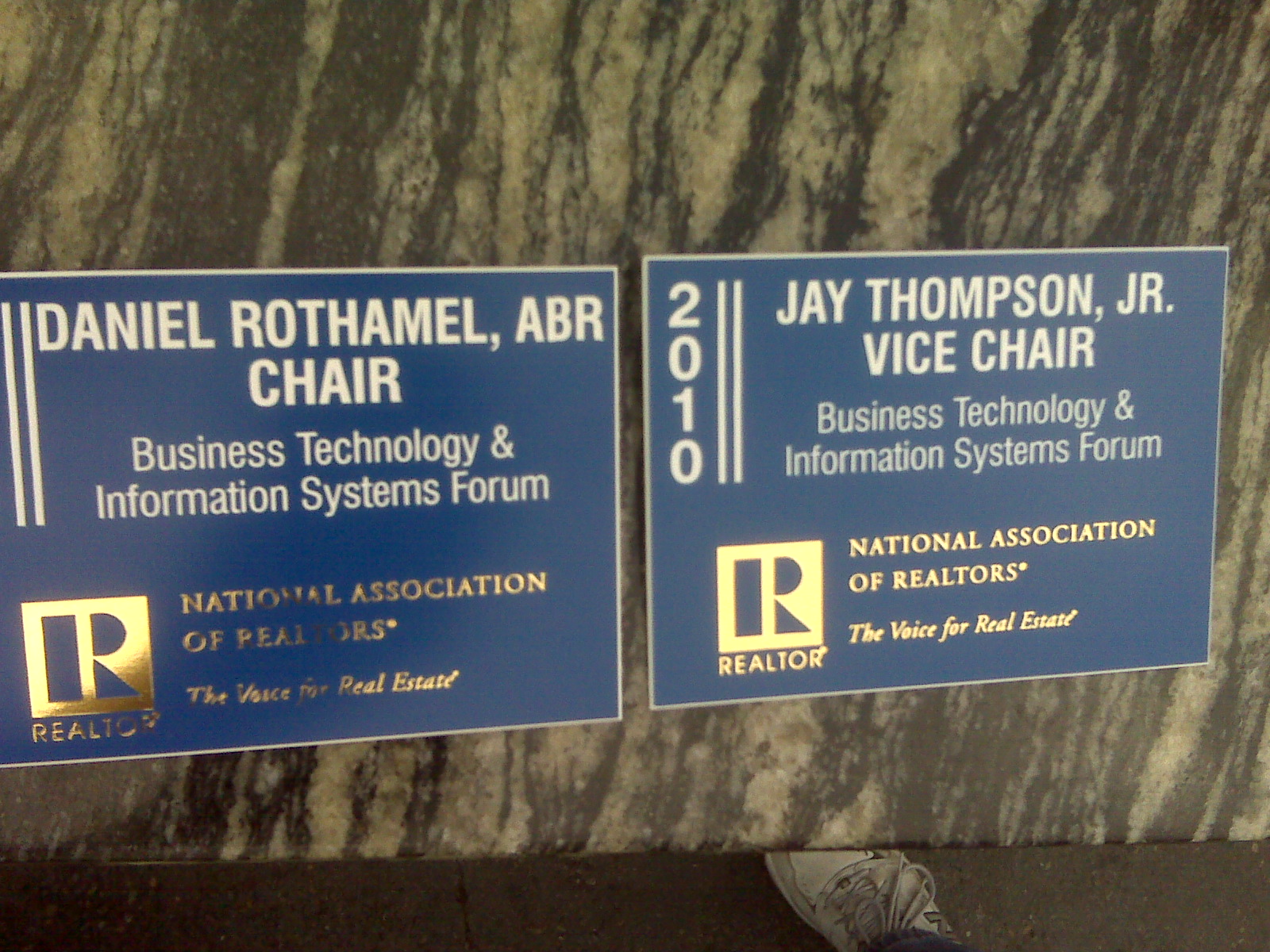This photograph captures two royal blue real estate business cards laid out on a granite countertop with gray stripes. The countertop and the polished concrete floor beneath it are both dark gray, providing a contrasting background for the cards. The cards, adorned with a thin white border, feature mostly white text along with some gold lettering. The card on the left belongs to Daniel Rothamell, designated as the ABR Chair of the Business Technology and Information Systems Forum, while the card on the right is for Jay Thompson Jr., listed as the Vice Chair of the same forum. Both cards prominently display the Realtor logo in gold, accompanied by the words "National Association of Realtors, the voice for real estate." The perspective of the photo reveals part of the photographer, who is dressed in blue jeans and white tennis shoes, adding a casual human element to the image.